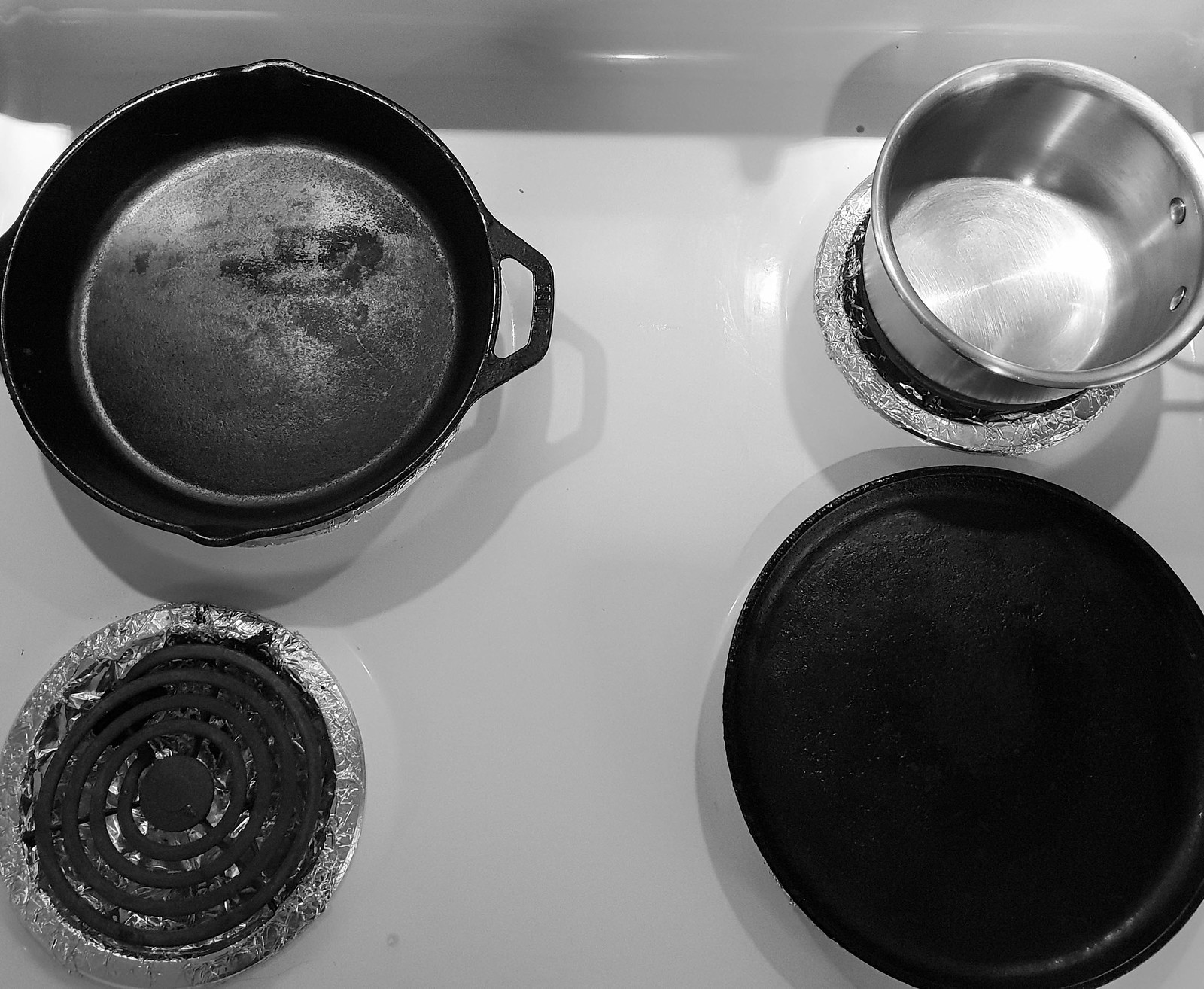The image is a detailed bird's-eye view photograph of a pristine white electric stove with four burners, each encased by characteristic black swirls and detailed in black and white. The stove is very clean, with the upper left burner cradling a cast iron pan. This cast iron pan features a small handle extending to the right and indents on both sides. Adjacent to it, on the upper right burner, sits a small, shiny silver pot with two rivets visible on the inside, hinting at the position of a handle. Moving to the bottom left, the burner there is empty but lined with aluminum foil, gleaming under the light. Finally, the bottom right burner is covered by an inverted black pie pan, possibly cast iron, serving as a makeshift cover. Shadows play over the stovetop, adding depth and intrigue to this meticulous kitchen scene.